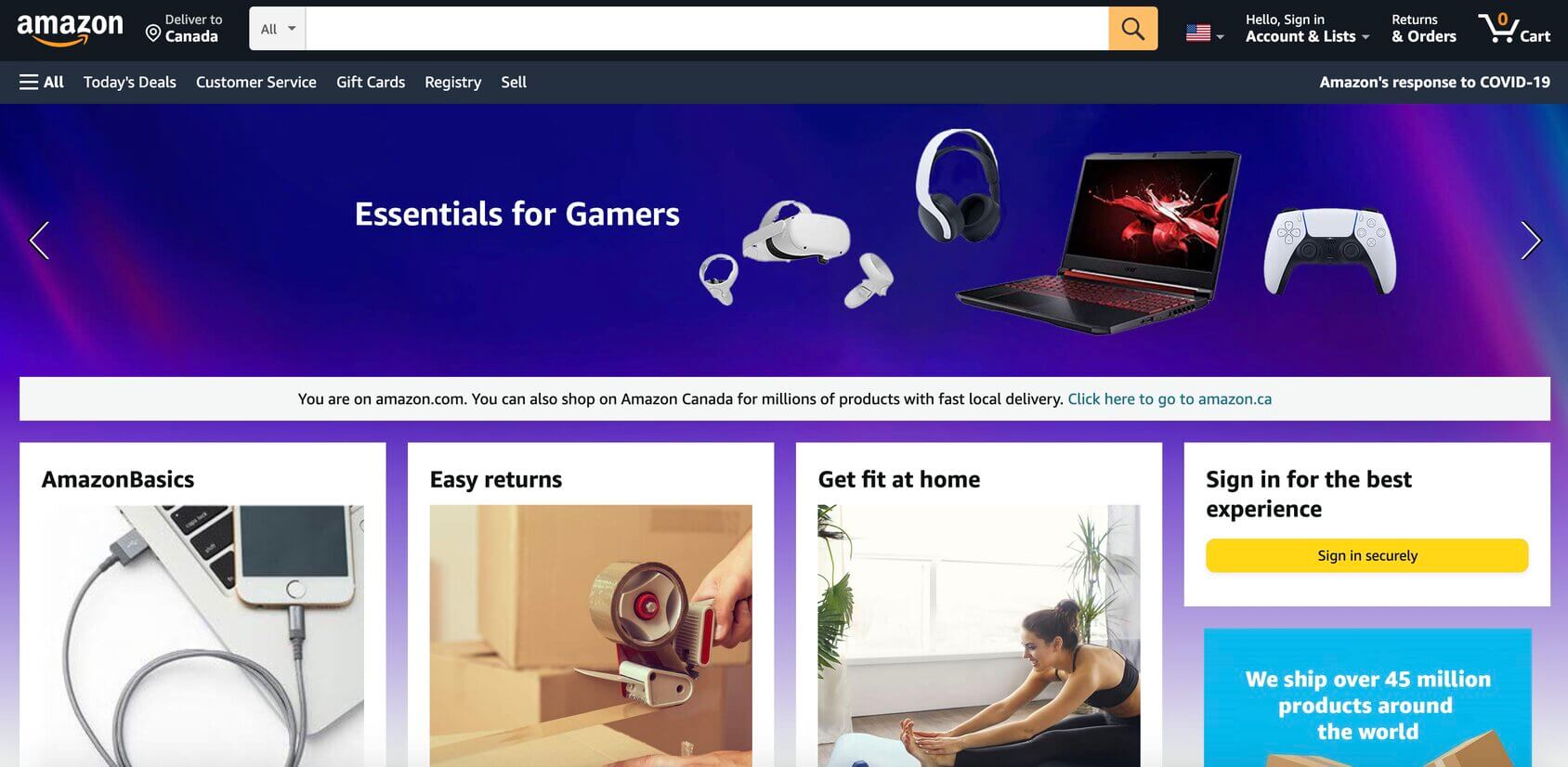Screenshot of the Amazon website. Across the top of the screen from left to right, there is a message indicating the site’s Canadian options. To the right, there's a search bar with a yellow search button. Next to it is an American flag icon. Following that, there's a greeting that reads "Hello, Sign in" with "Account & Lists" and a dropdown arrow beside it. To its right are the "Returns & Orders" link and a shopping cart icon for checkout.

Beneath this top navigation bar is a large blue rectangle featuring white arrows pointing left and right on opposite sides. In the center, white text reads "Essentials for Gamers." Displayed within this section are a pair of wireless earmuff headphones, a sleek red laptop, and what appears to be a gaming controller or a VR set.

Just below this section, there is a white rectangle spanning the width of the page. The text within reads, "You are on Amazon.com. You can also shop on Amazon Canada for millions of products."